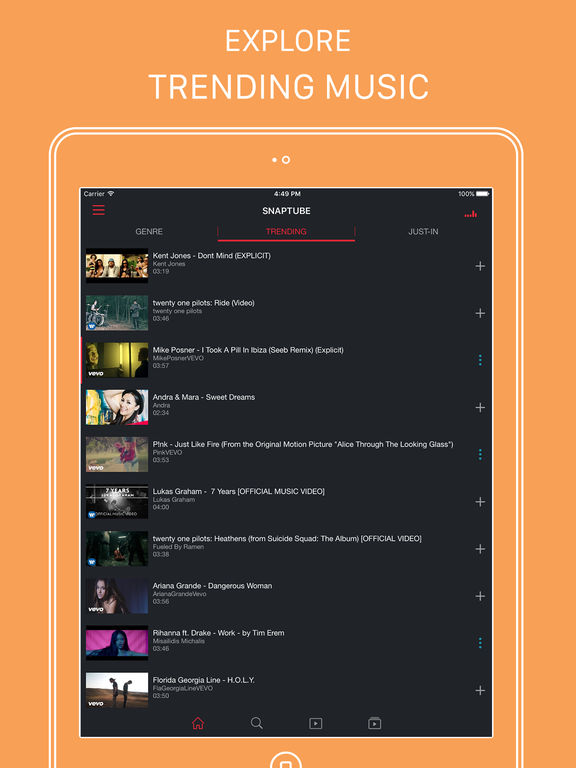The image showcases a web interface with a predominantly dingy orange background. The orange gradient starts at the top, extending down about two inches, and from the sides, it encroaches about one inch. At the bottom, the orange spans about a quarter inch. 

Centrally, at the top of the page, bold and large black capital letters spell out "EXPLORE." Beneath this, smaller text reads "Trending Music." 

On the left side of the page, there is a rounded-edge white border that frames the content. This border extends downward and then off the bottom of the screen. An orange trim follows the white border, and then another white border encapsulates the central black square area. This black square measures approximately three inches across and five inches vertically.

Above the black square, there is a small white dot encircled by a white outline, resembling a phone's notification icon. The top-left corner of the black square shows typical smartphone indicators: "Carrier," full Wi-Fi signal, and "4:49 p.m." in the middle, and a 100% battery indicator on the right, all in white text. Below "Carrier," three horizontal red lines are stacked. Underneath the time, "Snap Tube" is written in all capital white letters, with "Trending" in red and underlined beneath it. To the right, white text reads "Just In," and "Genre" is displayed on the left.

Below this section, there are ten clickable items arranged vertically. Each item has a thumbnail image from a video on the left, the video's name on the right, followed by the creator's name and the runtime. On the far right, a plus sign is displayed next to each video's information.

Across the bottom of the black square, there is a red home icon, a white search bar, a white play bar, and another play bar with a square behind it. Back in the orange section below, there is a half-circle and half-square graphic, partially within the circle.